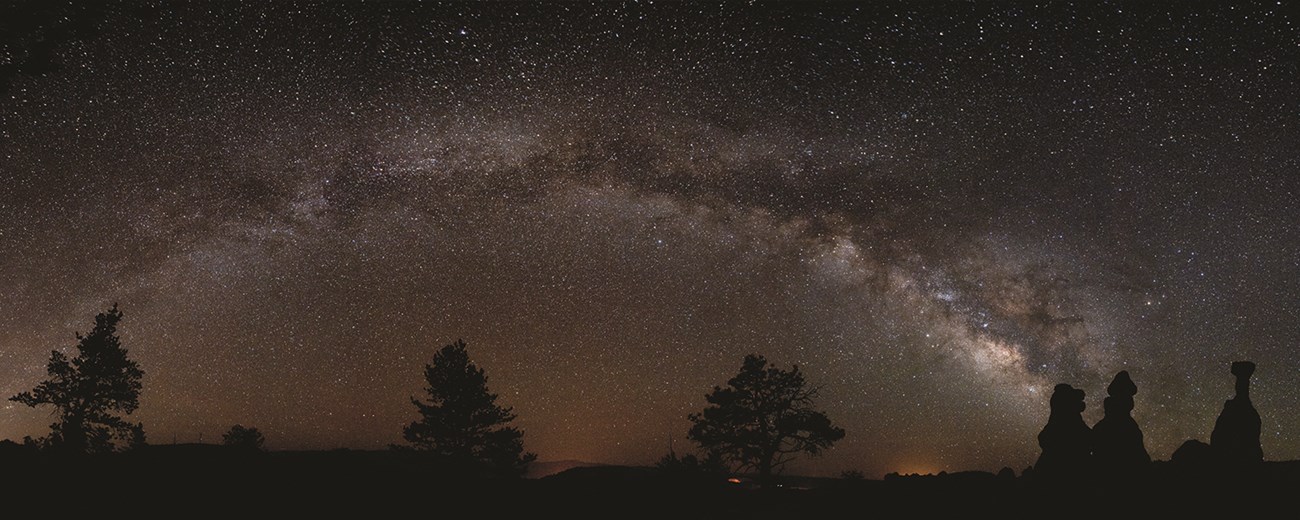This iconic photograph, captured by Keith Moore for the National Park Service, is titled "Starry Night Sky on Queens Garden Trail" and was taken in Bryce Canyon National Park. The image showcases a breathtaking night sky filled with countless stars, including a luminous arch of light that resembles a celestial rainbow, possibly the Milky Way. The sky, mostly dark with a soft gradient of brown and dark orange near the horizon, provides a striking contrast to the silhouettes of unique rock formations and three to four trees positioned on the bottom right side of the image. Adding to the mysterious ambiance, the stone formations have abstract shapes that resemble figures—one almost gorilla-like and another reminiscent of the character E.T., with a third appearing cone-headed. The combination of natural elements and the expansive, star-filled sky captures the ethereal beauty and grandeur of Bryce Canyon under the night sky.